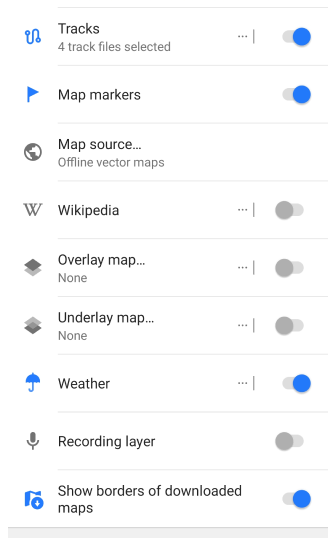The image is a screenshot taken from a back angle of someone's computer screen, showing a detailed interface with various selectable options and indicators related to map and track management.

On the left side of the screen, there is a vertical list entitled "Tracks" with four track files selected. Adjacent to the list is an array of icons that serve as visual guides or emblems for different functionalities. At the top, next to the "Tracks" heading, there's a small squiggly line or a sideways "S" symbol.

Just to the right of the icons, there is a series of on-off buttons. The first button, marked with a blue dot, is in the "on" position. Below this, a blue flag icon indicates the "Map Markers" section, which is also turned on. 

Further down, there is a "Map Source" section featuring an earth icon labeled "Offline Vector Maps," which is not activated (no indicator is present on the right side for this option). 

A "Wikipedia" section features a "W" icon, and its corresponding slider is turned off, shown by a gray indicator. Similarly, the "Overlay Map" and "Underlay Map" sections have their sliders turned off, indicated by gray sliders. 

Towards the bottom, the "Weather" section is turned on, the "Recording Layer" section is turned off, and the "Show Borders of Download Maps" option is turned on.